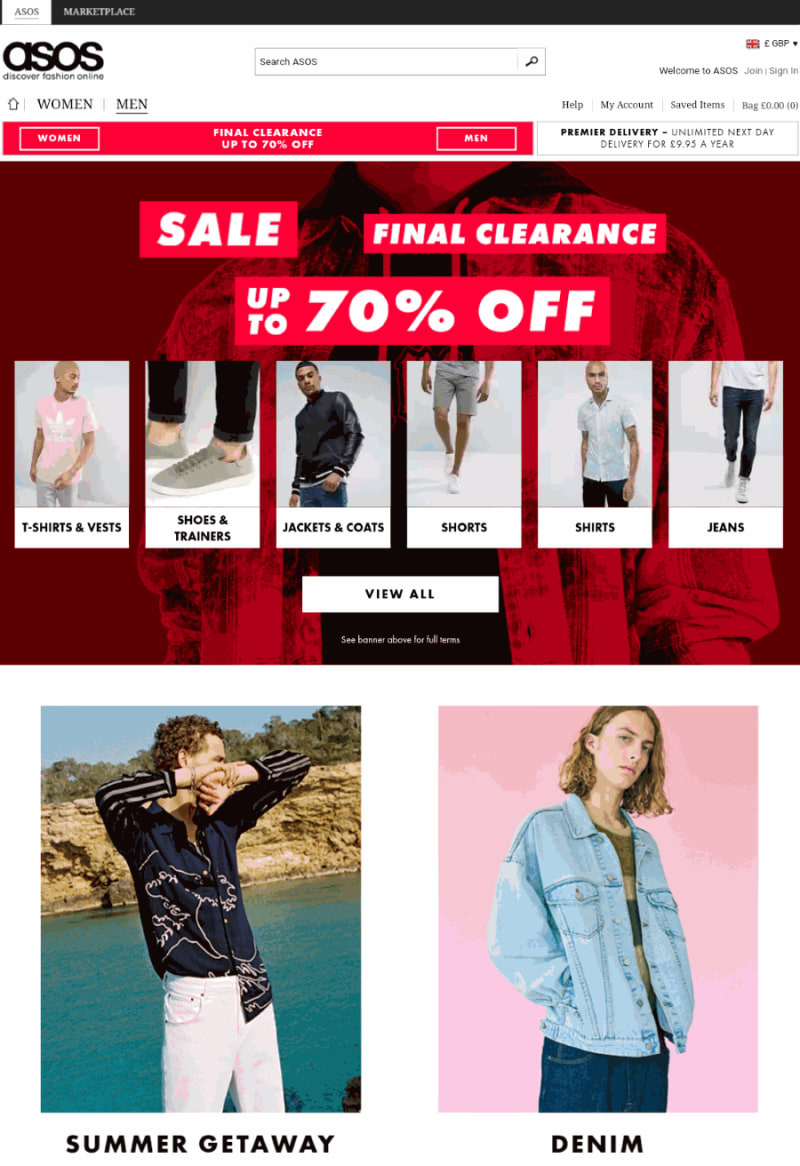The image features a clean white background with a small black line at the top left, followed by a black box displaying the "ASOS" logo. Next to it are the labels "Women" and "Men," accompanied by a search box. To the right, a prominent red box announces "Women: Final Clearance Up to 70% Off," and an adjacent section highlights "Men."

Below, a large image with a vivid red background states "Sale: Final Clearance Up to 70% Off," listing categories such as T-Shirts & Vests, Shoes & Trainers, Jackets & Coats, Shorts, Shirts, and Jeans. A "View All" button is visible beneath this list. 

There's also a small black box with fine print. The lower section of the image displays a photograph of a man standing in front of a scenic beach with the caption "Summer Getaway." Adjacent to this, a woman stands against a pink background wearing a denim jacket, with the word "Denim" beneath her. This image clearly delineates the sections for men's and women's sales.